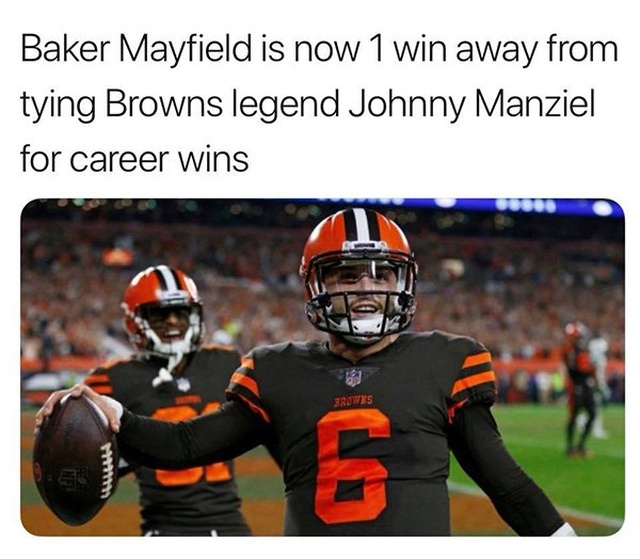In this detailed image, we see a lively scene on a football field. The bottom of the image features a flat, green, grassy field with painted white lines, resembling that of a football field. Positioned centrally are two football players from the Cleveland Browns. One, identified as Baker Mayfield, is a white player holding a football, while the other, an unidentified Black player, stands behind him with a smile. Both athletes are in an upright position, dressed in full football gear including helmets, and they seem to be celebrating, perhaps indicating a recent victory. Behind them, a blurred crowd makes up the background, illustrating that the setting is an outdoor stadium. Additional elements in the scene include blue lights, likely part of a scoreboard or advertisement typical to such venues. Dominant colors in the photo are orange, brown, white, red, beige, blue, purple, yellow, green, and black. At the top of the image, text reads: "Baker Mayfield is now one win away from tying Browns legend Johnny Manziel for career wins." The style of the photograph gives off a meme-like feel, possibly shared among fans and sports enthusiasts.